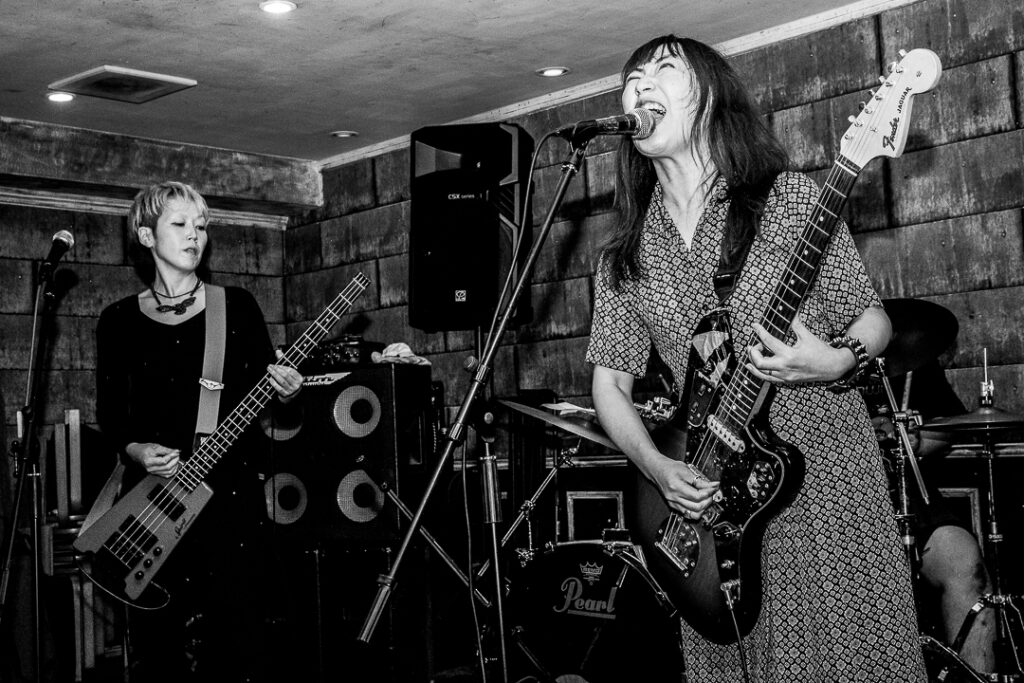This black and white photograph captures an intense live performance by a rock band featuring three members. Dominating the scene is an Asian woman with long dark hair, wearing a 1940s-style patterned dress, passionately singing into a microphone while playing a dark black Fender electric guitar. To her left stands another Asian woman with short bleached hair, dressed in black with a prominent necklace, focused on playing an electric bass. A microphone stands in front of her, though she does not appear to be singing. Partially obscured behind the lead singer, a drummer's leg is visible amidst a drum kit, hinting at their presence. The performance space is confined, with cinder block or concrete block walls and a smooth, low ceiling fitted with small puck lights. Amplifiers and various speakers are scattered in the background, contributing to the raw, intimate atmosphere reminiscent of a basement venue.